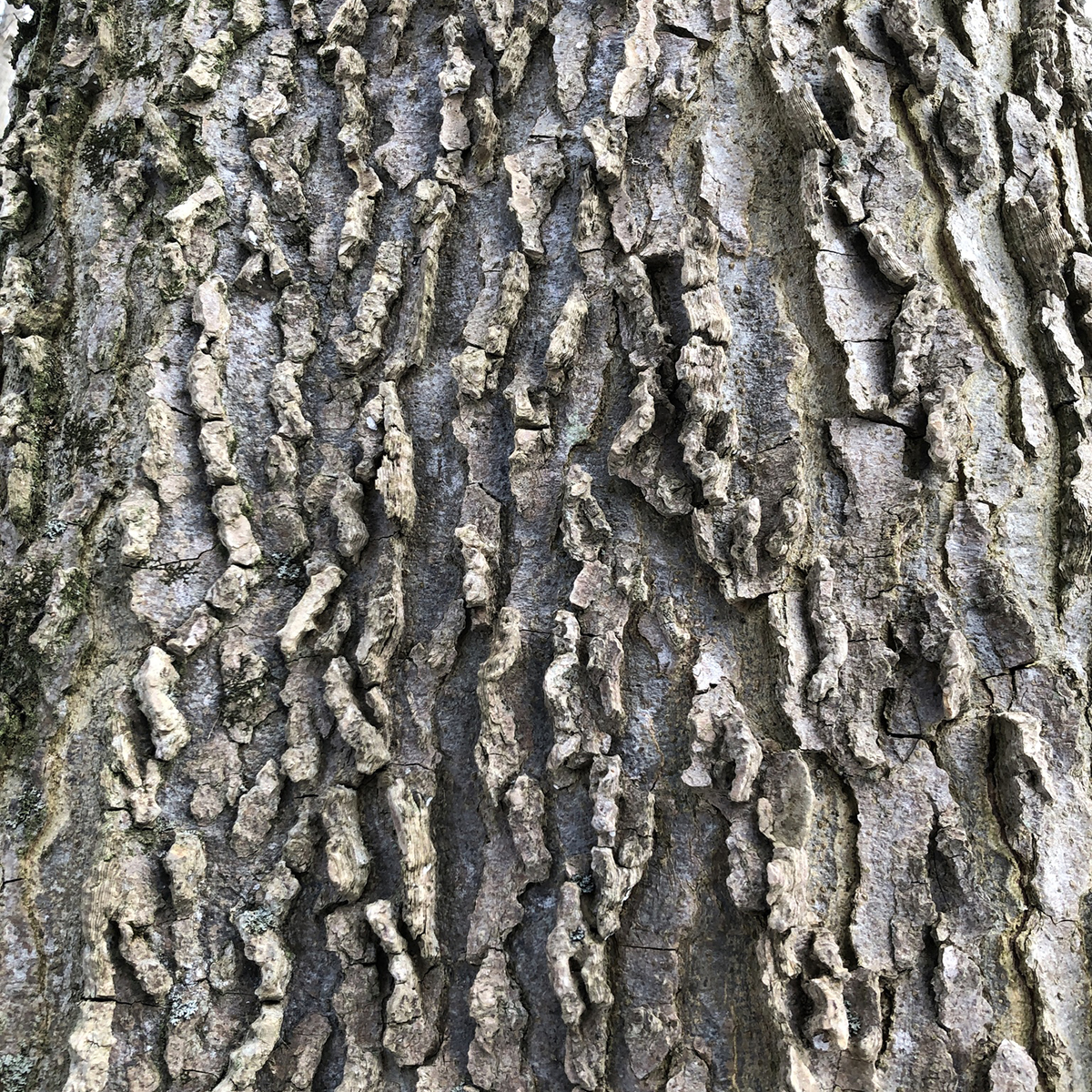This image is an extreme close-up of an old, but healthy tree trunk, highlighting the intricate textures of its bark. The photograph captures the deep ridges and valleys running mostly vertically along the surface. The bark appears largely intact with no signs of peeling or damage, indicating it has been undisturbed for quite some time. On the left side of the image, moss is visible, with varying shades of green adding a touch of color to the rugged bark. The sunlight illuminates the right side of the tree, casting subtle shadows that emphasize the bark's rough texture and the numerous gaps and cracks within it, including one notable crack about two inches from the bottom. The scene, likely captured on a partially overcast day, perfectly showcases the natural, untouched beauty of the aged tree.